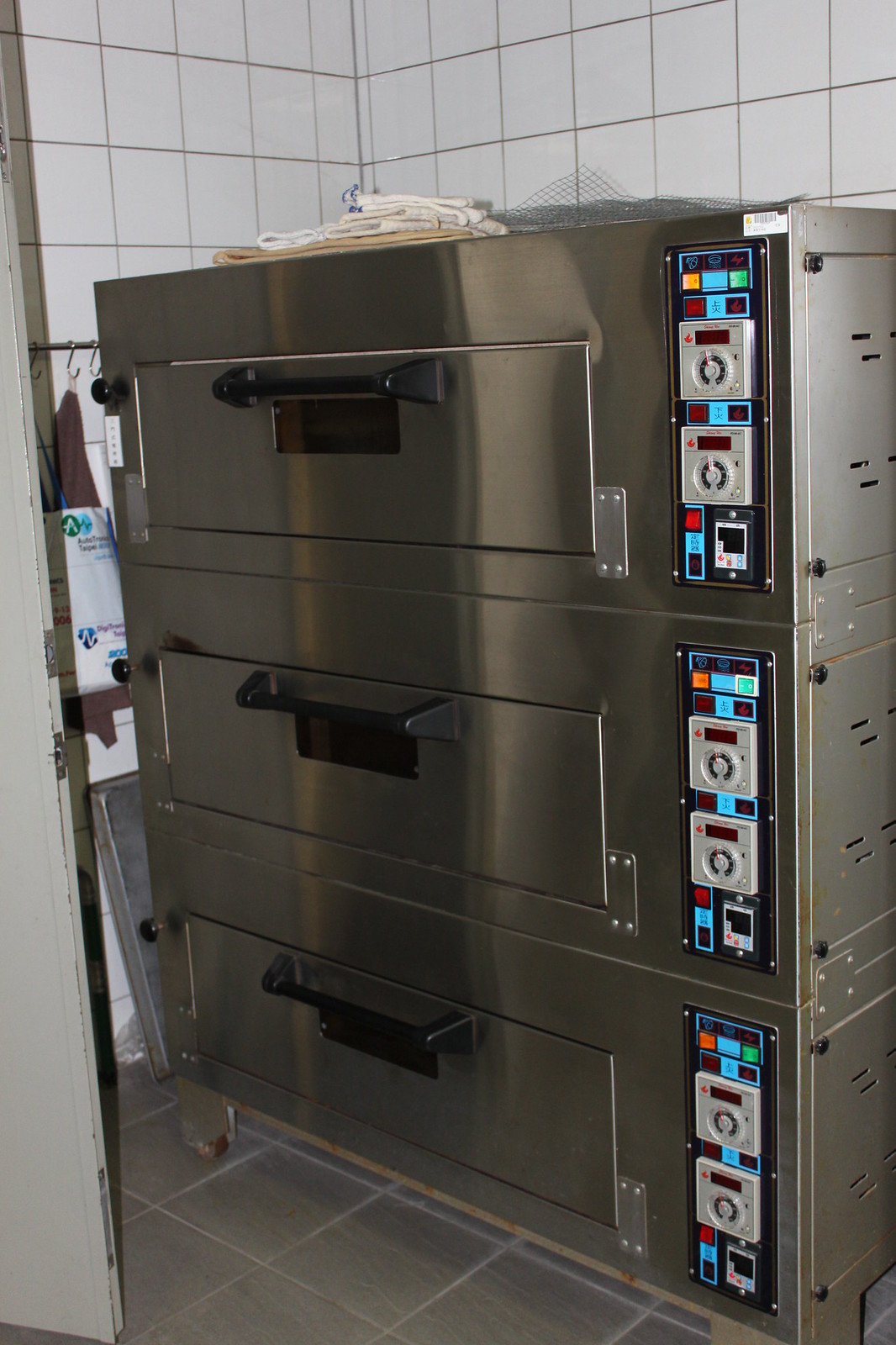This is a photograph of a stainless steel industrial machine, likely taken in a restaurant setting based on the presence of gloves and surrounding items. The machine appears to be composed of three vertically-stacked units, each resembling large drawers with black handles. Each unit is equipped with an array of controls on the right side, including multiple colorful buttons (orange, blue, green, red) and two dials, possibly for temperature or other settings. There are also digital readouts and displays, which might be used for configuring various parameters such as temperature or cook time.

Above the machine, there are various items including towels, a mat, and some plastic mesh or wire, indicating a utilitarian environment. The background features white tile walls with darker grout, giving a clean and structured appearance. To the left of the machine, there is an open door and some white boxes with unreadable green and blue lettering.

The machine itself suggests its use might be for cooking, perhaps for pizzas, given the industrial oven-like appearance and the possible temperature controls. The overall scene provides a glimpse into a well-organized, professional kitchen with a focus on functionality and efficiency.